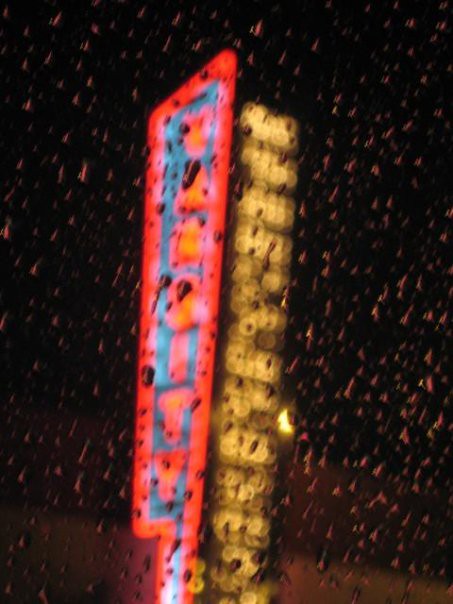The photograph captures a nocturnal scene observed from within a vehicle or possibly a house, with raindrops speckling the glass window through which the picture is taken. The raindrops on the window are the focal point, rendering the background out-of-focus. Beyond the rain-splattered glass, there are two illuminated billboard signs. 

The billboard on the left is striking with its vibrant red border and interior blue background, featuring red text that glows faintly in the blur. Meanwhile, the billboard on the right presents a more subdued yet elegant design with a black border and golden text that subtly contrasts against the dark night. The overall image emanates a moody atmosphere, capturing the quiet essence of a rainy night adorned by the mesmerizing glow of distant lights.